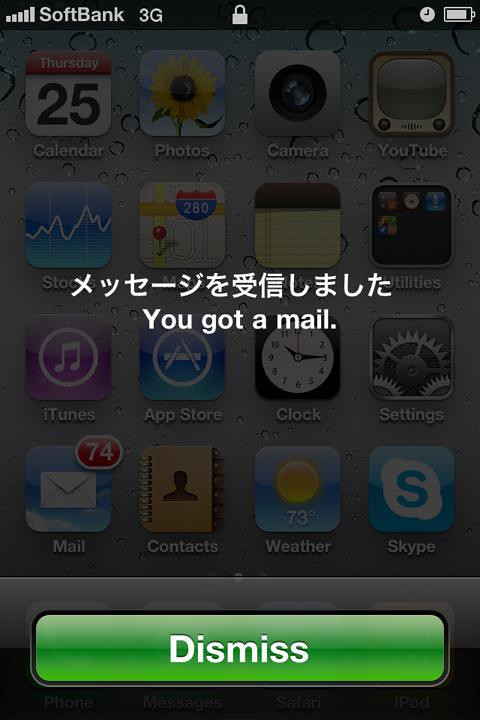The image is a screenshot of a locked iPhone home screen with a SoftBank service provider. The top bar displays five signal bars and 3G connectivity, alongside battery life and a lock icon. The background features a grayish, dewdrop design, and there is a prominent notification in the middle with white Chinese characters, followed by an English text saying "You got a mail." A green rectangle at the bottom with "Dismiss" in white text is visible, indicating an option to clear the notification. The home screen reveals several classic app icons, including Calendar (showing Thursday the 25th), Photos, Camera, YouTube, Skype, Mail (noting 74 new messages), Contacts, Weather, Stocks, Maps, Notes, Utilities, iTunes, App Store, Clock, and Settings. The overall design and app logos suggest that this screenshot is from an older model of an Apple iPhone.